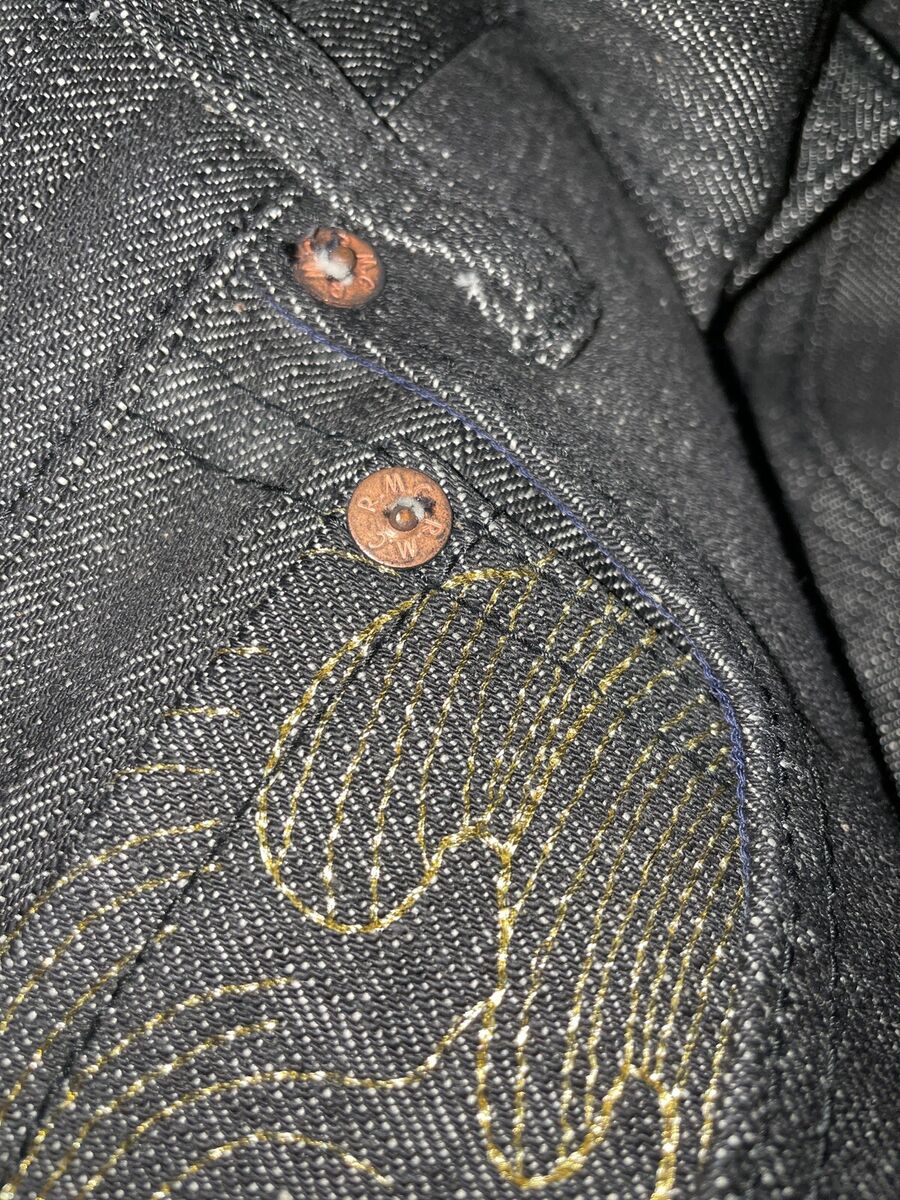This image depicts a close-up of a dark gray denim item, most likely a pair of jeans, characterized by its detailed texture and various stitching patterns. The denim fabric is dark gray, adorned with numerous small white speckles that give it a sequin-like appearance. The focus of the image seems to be on the back of the jeans, highlighted by one visible belt loop and a pocket. The pocket stands out with a light yellow design resembling part of a clover, intersected by horizontal gold lines. There are two rust-colored buttons, one on the pocket and another near the belt loop, both displaying the inscription "P.M.C."

In addition to the gray fabric, there is notable blue stitching around certain areas, likely the main pocket or where a zipper might start, and black stitching along other edges. The intricate details include rivets, which appear worn and carry the same "P.M.C." inscription, reinforcing the utility and durability of the garment. The overall impression is of a well-worn, meticulously crafted piece of denim clothing, rich in both functional and decorative details.